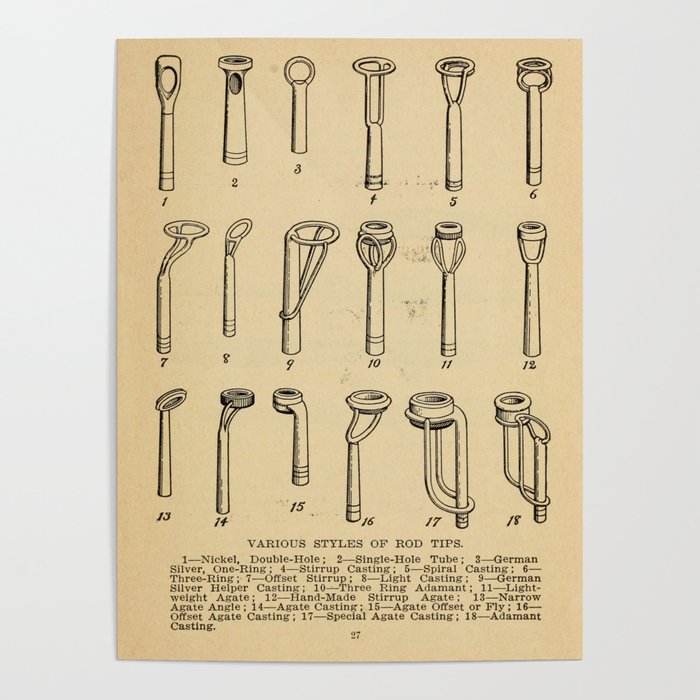The image is a detailed, aged book page with a subtly yellowed backdrop, displaying 18 black-and-white illustrated rod tips arranged in three rows. The page is numbered 27 at the bottom. The rod tips vary in size and design, each meticulously drawn in ink. Below the illustrations, a small paragraph identifies each rod tip, listing them numerically from 1 to 18. The descriptions include: 

1. Nickel double hole
2. Single hole
3. German silver one ring
4. Stirrup casting
5. Spiral casting
6. Three-ring
7. Offset stirrup
8. Light casting
9. German silver helper casting
10. Three-ring adamant
11. Light wing agate
12. Handmade stirrup agate
13. Narrow agate angle
14. Agate casting
15. Agate offset fly
16. Offset agate casting
17. Special agate casting
18. Adamant casting

Each number corresponds to an illustration above, providing a clear visual reference for each type of rod tip. The simple white background ensures the focus remains on the detailed imagery and text. The page title "Various Styles of Rod Tips" further clarifies the content, making it a comprehensive guide presumably related to fishing equipment.